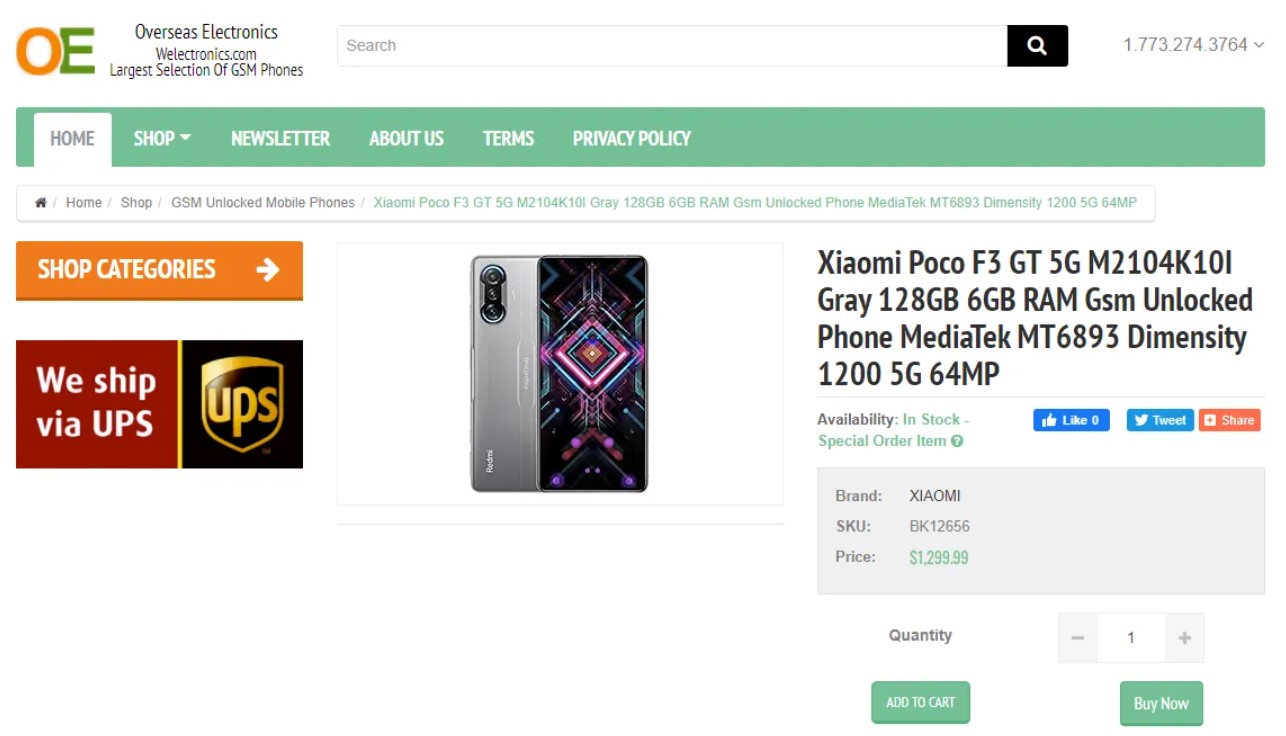The image depicts a website screen from "Web Electronics," a retailer specializing in GSM phones. Dominating the header are the brand's logo, featuring an orange "O" and a green "E," both capitalized, followed by the company name "Overseas Electronics" and the website "webelectronics.com." Below the logo, the site proclaims it offers the "largest selection of GSM phones." A search bar with a magnifying glass icon is prominently positioned for easy navigation. 

A navigation menu spans across the top, containing links labeled: "Home," "Shop," "Newsletter," "About Us," "Terms," and "Privacy Policy." 

The main focus of the screen is a highlighted product listing for the "Xiaomi Poco F3 5G." The detailed listing includes the product name "Xiaomi Poco F3 5G, M2104K, 101 Gray," with specifications such as "128GB storage" and "60GB of RAM." The phone is described as a "GSM unlocked phone" and features the "MediaTek MT6893 Dimensity 1200 5Q64MP" chipset. The product is identified by the brand "Xiaomi" and SKU "BK12656." The listed price is "$1,299.99," with options to "Add to Cart" or "Buy Now."